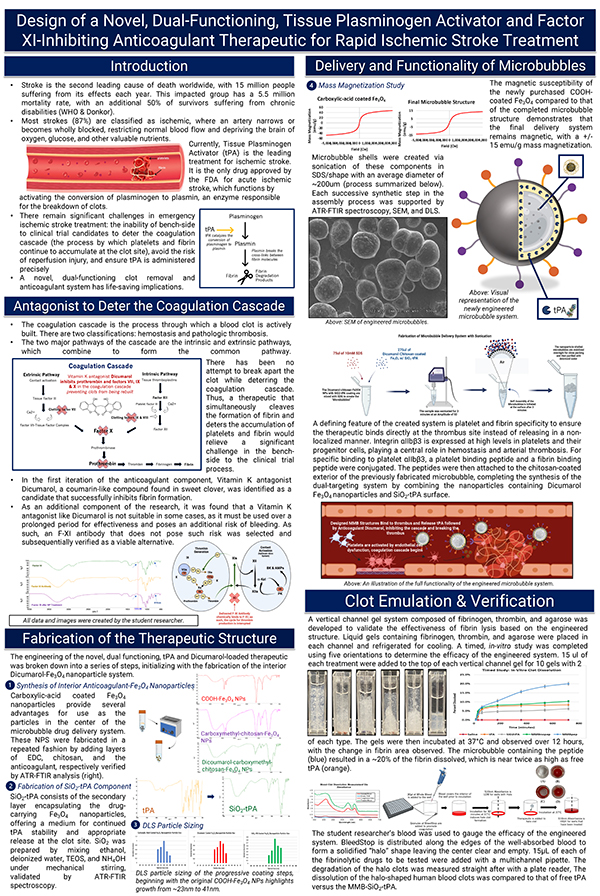The image is a digitally synthesized infographic titled "Design of a Novel Dual Functioning Tissue Plasminogen Activator and Factor XI Inhibiting Anticoagulant Therapeutic for Rapid Ischemic Stroke Treatment," prominently displayed in white text on a blue background at the top. The primary background of the image is white, with text primarily written in black. There are multiple sections, each introduced by subtitles in white text on blue backgrounds, detailing different aspects of the therapeutic design. 

The top left section, under "Introduction," includes paragraphs and images, possibly of human veins. Directly beneath is the section titled "Antagonist to Deter the Coagulation Cascade," featuring more text and pictures related to this aspect. Following this is "Fabrication of the Therapeutic Structure," which also includes text along with various graphs and charts. 

On the top right, another section titled "Delivery and Functionality of Microbubbles" incorporates graphs, synthesized images, and explanatory text focusing on this innovative delivery method. Below this, the section "Clot Emulation and Verification" includes simulated images, additional graphs, pictures, and further descriptive text to verify the effectiveness of the therapeutic. The organized layout with detailed visuals and comprehensive text offers an in-depth overview of the innovative stroke treatment process.